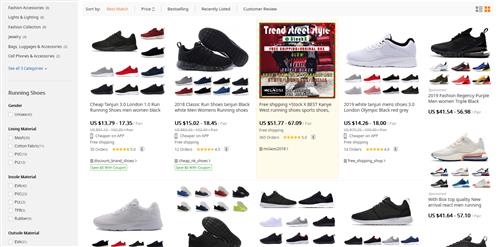The image depicts a screenshot from a sales-focused website. At the top of the page, there are six small, unreadable buttons likely for navigation or additional functionalities. Running along the entire left side, a dedicated filtering panel features multiple empty check boxes labeled with text, suggesting options to refine the product search results.

The main content area displays several product listings, all of which appear to be shoes. Each listing includes a clear photograph of the shoes, accompanied by a title beneath it. Prices are indicated for each product, with the first listing showing a price range from $13.79 to $17.35, presumably in US dollars. Product reviews are also visible, represented by star ratings, with the first four listings clearly displaying their ratings. Further down, some listings have truncated titles and partially visible star ratings, indicating a larger list of product options that extends beyond the visible portion of the screenshot.